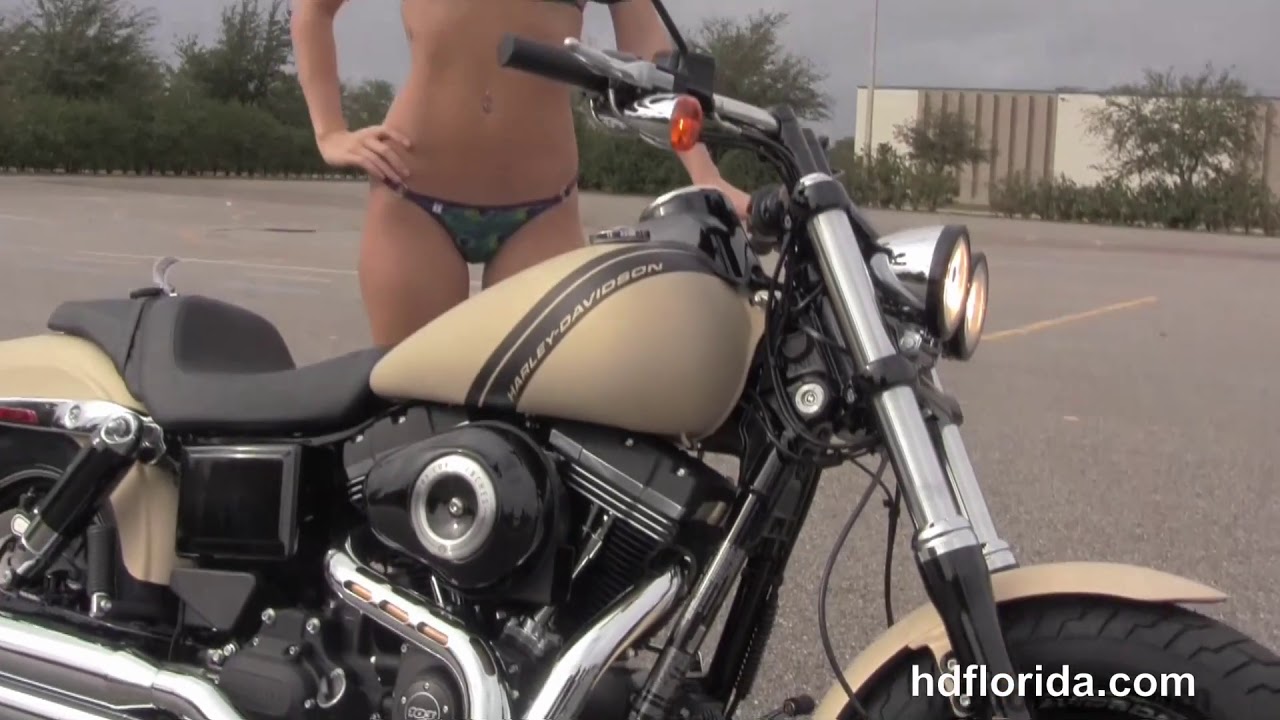The image is a high-definition photograph of a Harley-Davidson motorcycle and a woman standing behind it, set in a gravel parking lot with orange and yellow parking space stripes. The motorcycle, with its right side facing the camera, prominently features a gas tank with "Harley-Davidson" inscribed on a black strap. The gas tank, front fender, and back fender are a light cream color, while the rest of the motorcycle includes black and chrome elements, such as chrome-colored front forks, handles, lights, and exhaust. The seat is black. The bottom left corner of the image includes the text "HDFLORIDA.COM."

Behind the motorcycle, a woman is standing in a bikini, with the camera capturing her from the chest down to her feet. She has light skin, a slim build, and is wearing camouflage-patterned bikini bottoms. Her right hand rests on her hip while her left hand touches the motorcycle. The background includes a cloudy gray sky, a row of dark green trees, and a tall building with white sections on both sides and a brown section in the middle, partially obscured by two trees and a metal pole. The image captures a blend of rugged motorcycle aesthetics with a casually posed figure in an industrial outdoor setting.